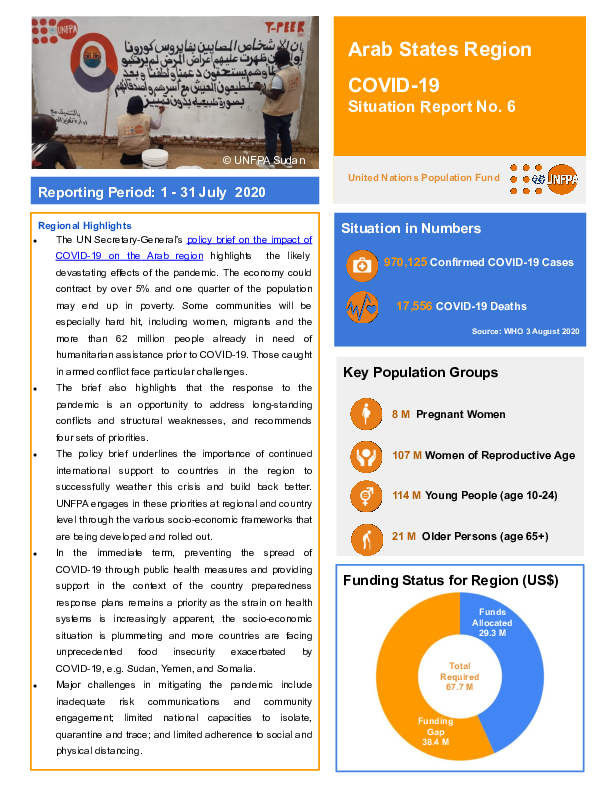**Descriptive Caption:**

In the foreground of the image, a white wall serves as the backdrop for various textual and graphical elements. To the left, there is a picture of people writing a message in Arabic, painted in black against the white wall.

Adjacent to this image, an orange rectangle features the text "Arab States Region" in white. Below this, another line reads "COVID-19 Situation Report" followed by "0.6." 

To the far left, a blue rectangle contains white text stating "Reporting Period: 01-31 July 2020." Beneath this, there is an orange-bordered white rectangle containing key highlights. At the top, a blue headline reads "Region Highlights." 

Below this headline, several bullet points provide detailed information:

1. **UN Secretary General's Policy Brief:** This brief discusses the impact of COVID-19 on the Arab region, highlighting potential devastating effects. The economy could shrink by over 5%, with up to one-quarter of the population falling into poverty. Particularly vulnerable groups include women, migrants, and over 62 million people already in need of humanitarian aid before the pandemic.

2. **Opportunity for Addressing Conflicts:** The policy brief suggests that the pandemic response could be a chance to tackle long-standing conflicts within the region.

3. **Continued International Support:** It emphasizes the significance of ongoing international aid to help countries in the region manage the crisis.

4. **Immediate Priorities:** Preventing COVID-19 spread through public health measures and providing support within country preparedness frameworks remains crucial.

5. **Major Challenges:** The final bullet point notes substantial obstacles in mitigating the pandemic, including inadequate risk communication and community engagement.

To the right, another blue rectangle is labeled "Situation in Numbers." In orange, it displays "970,125" as the count of confirmed COVID-19 cases, and "17,556" in orange indicates the number of COVID-19 deaths.